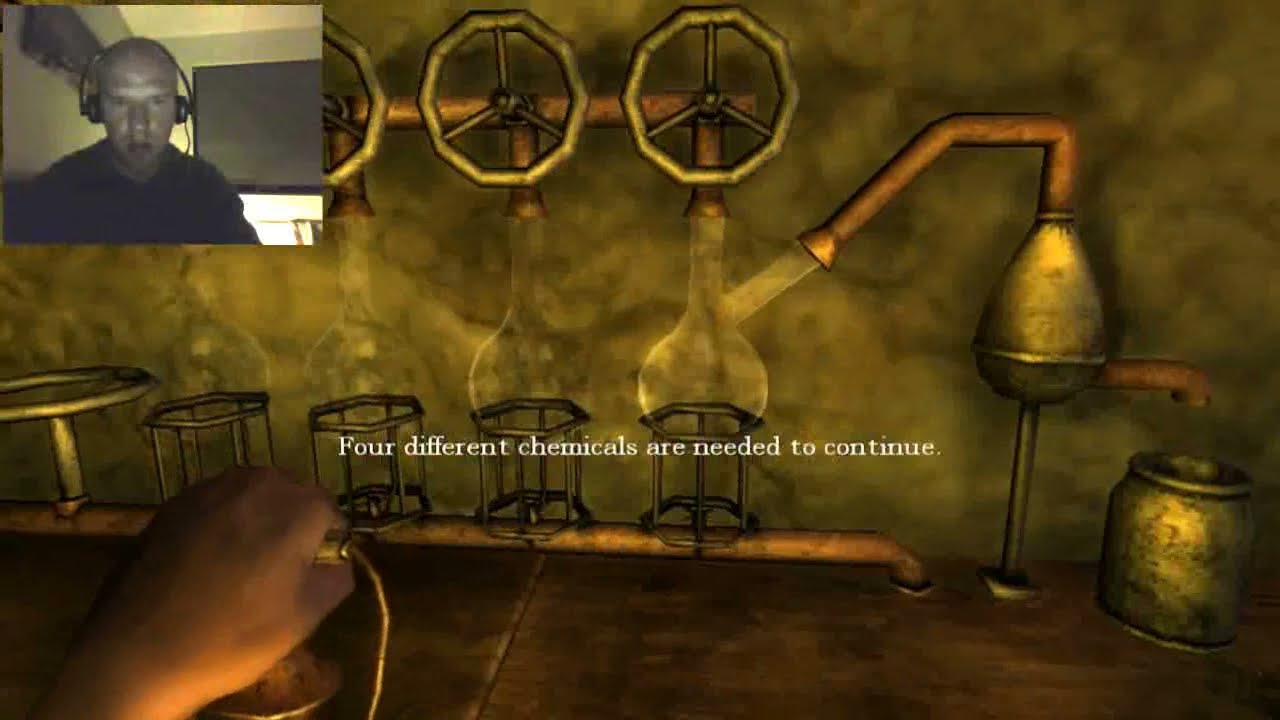The image is a detailed screen grab, likely from a video game, featuring a hybrid of a dark, shadowy room illustration and a webcam feed. The background illustration shows an open book with vintage ink drawings of doorways and arches, smeared ink, and illegible handwriting. A light green feather quill lies across the book's bottom right corner. The webcam feed in the upper left corner depicts a man with headphones and a microphone, probably reading the text on the screen. This inset is somewhat poor in quality, partially obstructing the white text on the image. The visible text includes crucial information for the game: "Key for the wine cellar of organic tissue blocks the path to the refinery. Can it be? Chemical ingredients have been moved from the laboratory to the wine cellar. Evidence in the laboratory has revealed that combining four chemicals can create a powerful acid." The eclectic combination of a video still, text overlay, and detailed illustration indicates a rich, narrative-driven game environment.